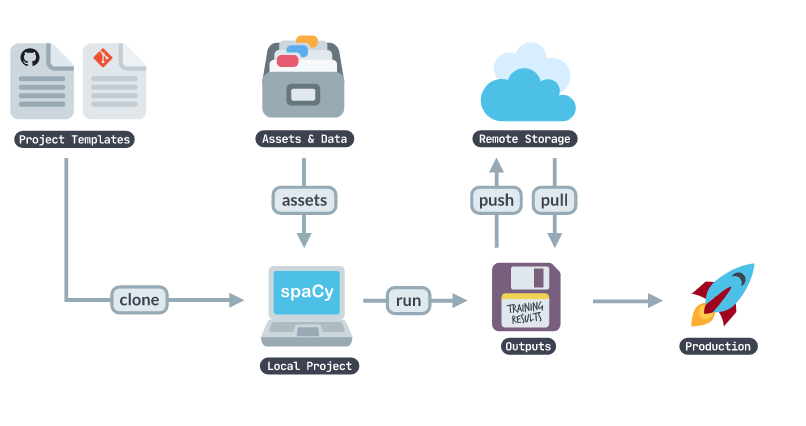This meticulously detailed timeline illustrates the step-by-step workflow of a program. At the top, we begin with the "Project Template," symbolized by two pieces of paper. A vertical line descends from this point, marked halfway down with the word "Clone," before branching off to the right towards the "Local Project." This local project is depicted by a laptop displaying the word "SPACY."

Above the local project, we see a file cabinet brimming with folders, labeled "Assets and Data," and an arrow directs from the cabinet downwards to the local project, implying that these assets are being transferred to it. 

Next, an arrow labeled "Run" extends from the local project towards an icon of a floppy disk, representing "Outputs." This signifies the execution phase where the project's assets and templates are being processed to generate outputs.

From the outputs, an arrow marked "Push to Cloud" points to "Remote Storage," indicating that the processed outputs are being uploaded for cloud storage. Additionally, another arrow loops back from the remote storage to the outputs, annotated with "Pull," representing the retrieval of data from the cloud back to the local system.

Lastly, an arrow labeled "Production" leads from the outputs to a rocket ship icon, symbolizing the final deployment stage where the complete project is launched into production.